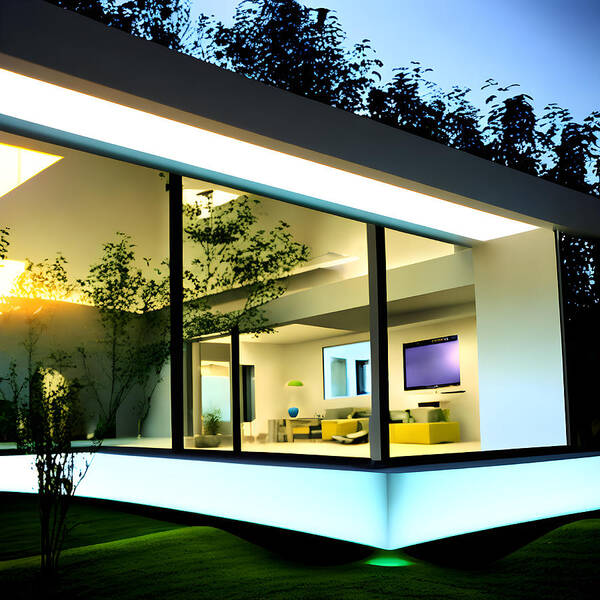This image is a detailed 3D color illustration resembling those created in apps like 3D SketchUp. It captures an outdoor scene at dusk, showcasing a modern, minimalist home with a strikingly white exterior and sleek black trim. The architectural design is geometric with a flat roof and wide, open glass windows that offer a clear view into the house. 

Inside, there is a living room characterized by its clean lines and minimalist decor. A large, purple flat-screen TV is mounted on the wall, accompanied by a mirror next to it. Below the TV, a greenish-yellow couch completes the cozy setup. To the left of the mirror, a table adorned with a bluish-green lamp adds a splash of color to the space. 

Additionally, tall plants are visible, either inside the living room or just outside. The green lawn surrounding the house is slightly illuminated, contributing to the calm ambiance as the sky transitions from light to dark blue. Black silhouettes of trees rise above the roofline, enhancing the serene, twilight atmosphere. The structure also features a distinctive porch section on the right side, with a glowing green light underneath the central post nearest to the viewer. The overall scene is a meticulously crafted representation of modern living, with both interior and exterior elements seamlessly integrated.